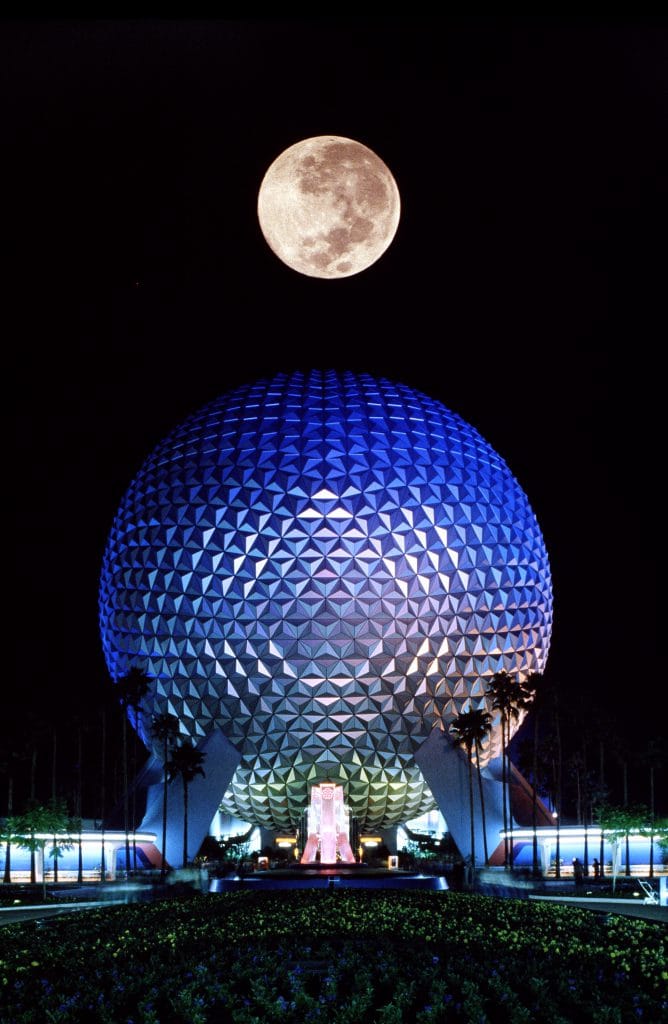This nighttime photograph captures the striking scene at Disney World’s Epcot Center. Dominating the image is the large spherical building known as Spaceship Earth, reminiscent of a giant golf ball with its intricate diamond-shaped facets. The structure features a luminous blue hue at the top, transitioning to silver and then reflecting green near its supporting pillars, suggesting a highly reflective material rather than fixed colors. Flanked by low buildings and tall palm trees, the spherical building stands out against the dark night sky. The full moon, positioned directly above the sphere, shines brightly with visible lunar details, adding a surreal and almost staged quality to the scene. The ground in the foreground appears illuminated, possibly by lights along the lawn that hosts various plants, further enhancing the magical ambiance of the setting.